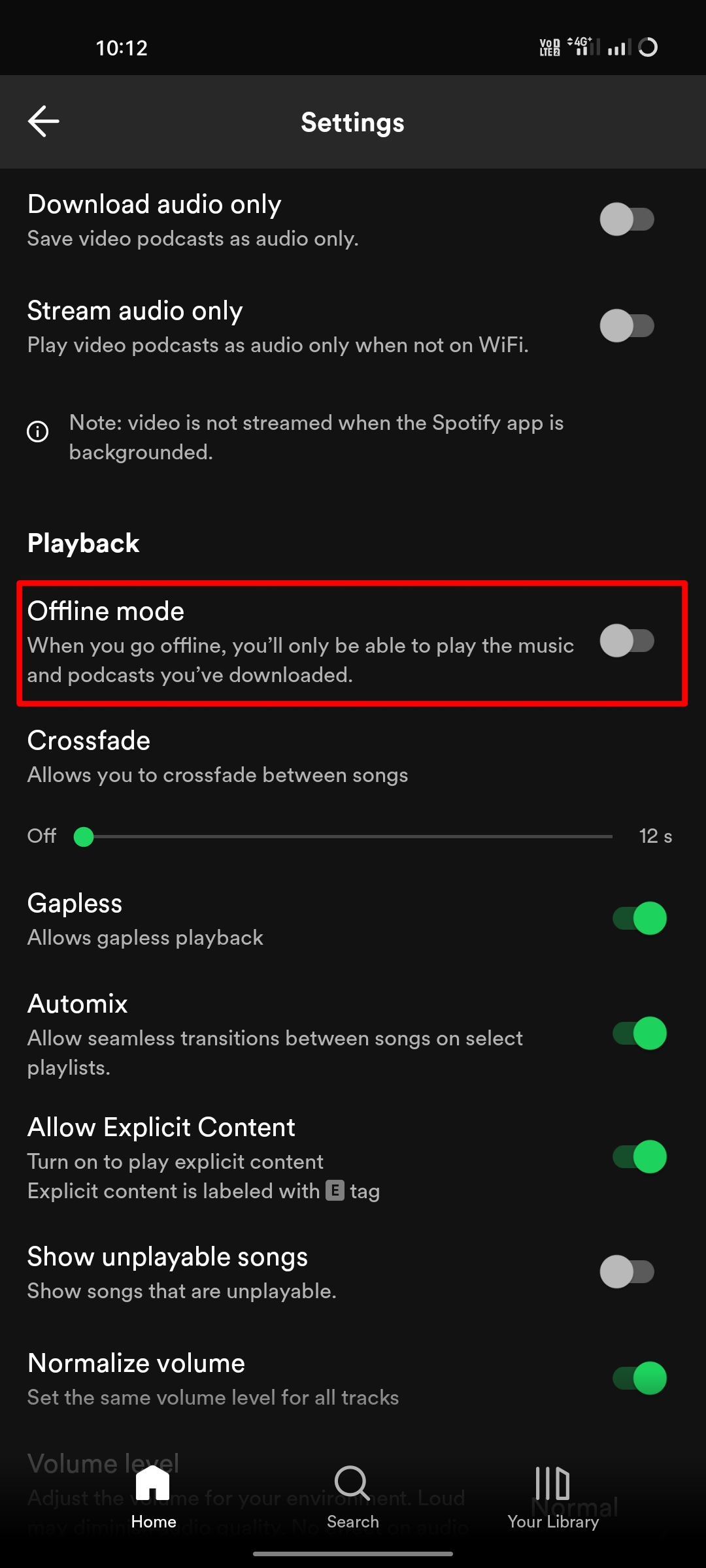User navigates through the Spotify app settings to optimize audio playback. The signal strength indicator fluctuates between 10 and 12, suggesting a near-full connection. The user highlights the 'Download Audio Only' option within the settings, saving VOD podcasts exclusively as audio files to save bandwidth. They ensure streaming of podcasts in audio-only mode, avoiding data use on Wi-Fi by toggling off video streaming. A red border surrounding the screen indicates 'Offline Mode,' notifying that only downloaded music and podcasts can be played offline.

Various toggles including 'Crossfade' are adjusted for smooth transitions between songs. The 'Auto-Mix' feature is enabled for seamless playlist transitions, and 'Explicit Content' is turned on to allow playback of mature content. Video playback options are managed, ensuring predictable file naming with 'Normalize Filename' for consistent labeling of downloaded files. The user’s journey ends navigating back to Spotify's main sections—Home, Search, and Library—tailoring the app for a streamlined, efficient audio experience.